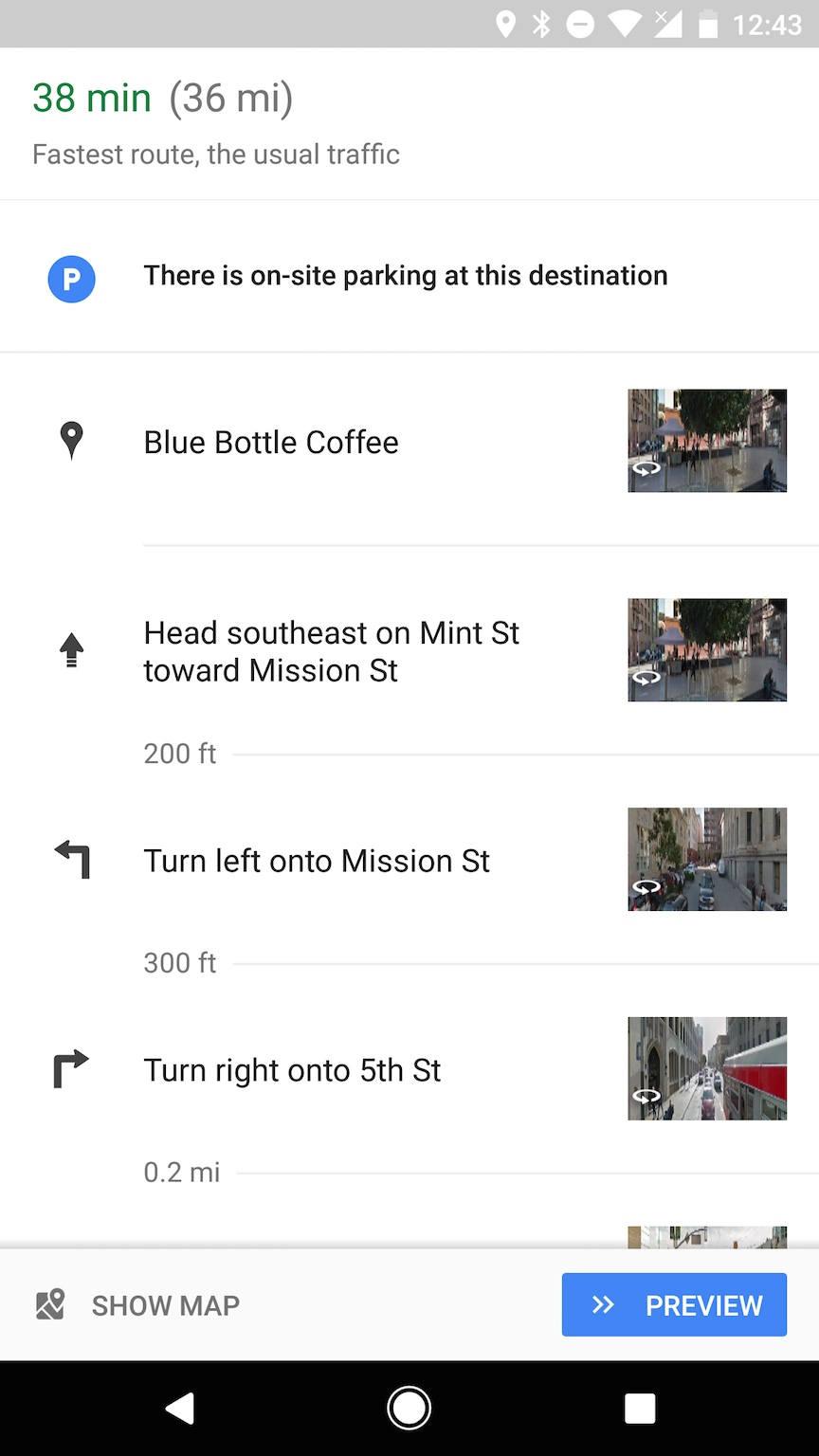A screenshot from a cell phone display shows various on-screen elements:

- At the top, there is a gray status bar containing several icons: a location pin, Wi-Fi symbol, a star with a gray center, full Wi-Fi bars, full cell coverage with an "X" over it, and a battery icon indicating 25% charge remaining. The time displayed is 12:43, with the numbers in black text against a white background.
- Below the status bar, a section shows "38 minutes of 38 minutes" with "36m" (indicating 36 miles) in parentheses, followed by "Fastest route, usual traffic."
- A white box surrounded by a blue border contains the message "There's on-site parking at this destination," accompanied by a black location pin and the text "Blue Bottle Coffee." Next to it, a street view image shows a small white shop.
- Directions are provided sequentially:
  1. "Head southeast on Mid Street towards Mission Street" — an upward-pointing arrow, followed by "200 feet" in gray text.
  2. "Turn left onto Mission Street" — a left-turn arrow, with "300 feet" in gray text on the left.
  3. "Turn right onto 5th Street" — a right-turn arrow, showing "0.2 mi" (0.2 miles) in gray text, accompanied by an image of two different buildings and a bus driving by.
- At the bottom, options to "Show map" (with a map icon) on the left and "Preview" (white text on a blue button) on the right are displayed.